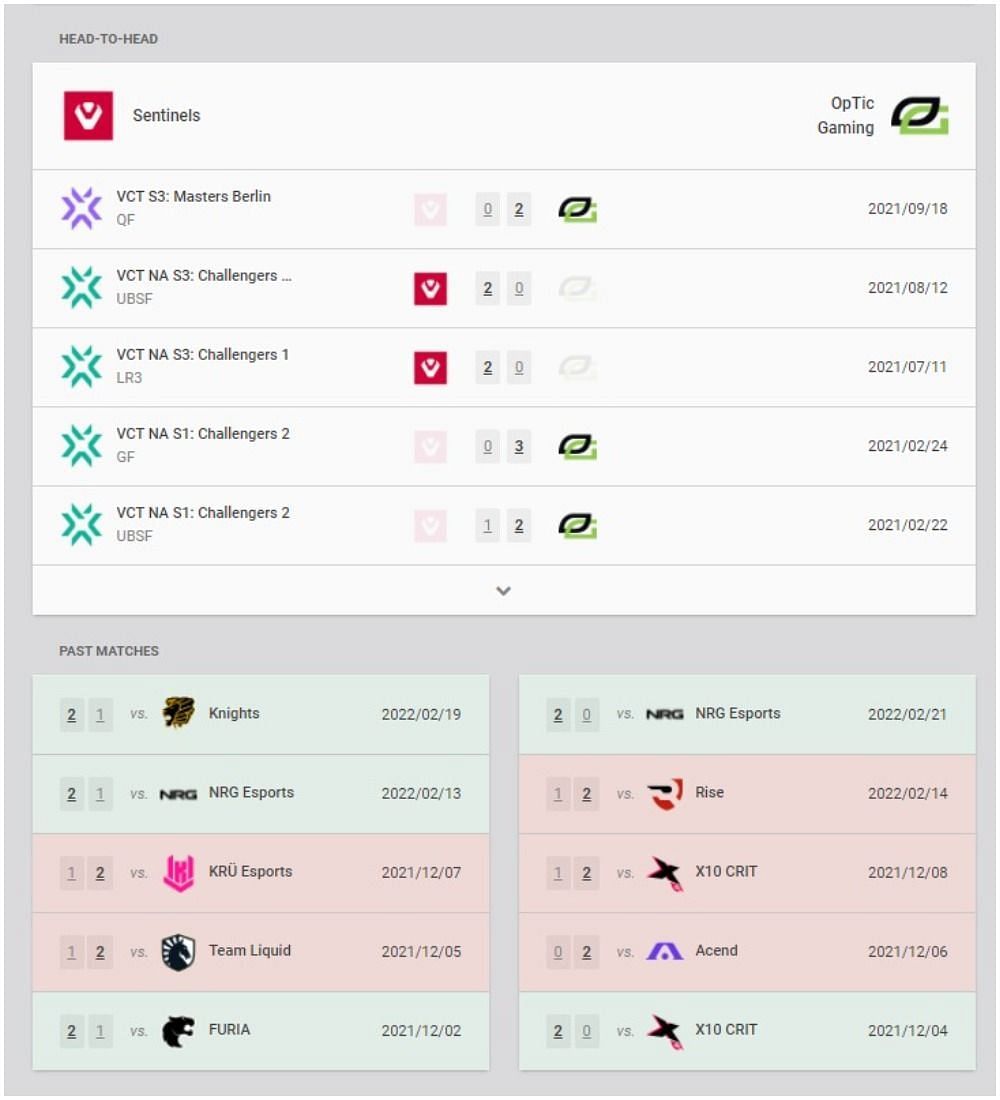In a high-stakes showdown, various teams compete head-to-head in a series of talk shows, including Riot Squares, Sentinels, Puck, Big Gaming, and Lee's. VCT SC Masters Berlin Quarter-Finals are highlighted with detailed stats: Graves at 0-2, Twins at 0-1, and multiple sets ranging from 0-9 to 0-13. In the VCT Nades Season 3 Challengers, VSF showcases a record of 2-0, Twins at 0-1, and multiple sets including 0-12 and 1-2. Sentinels emerge as the victors in this segment.

Continuing, VCT Nades 1-Challenger and 2-TF display scores of 0-3 and OpTicGaming at 1. During the VCT Nades 1-Challenger event, OpTicGaming secures a win. Further, Passages plays out with a 2-1 victory against the Knights, 22-2, followed by evenly matched sets against NRG Esports, concluding at 2-1. Other notable results include a 1-2 loss to KRU Esports and a 1-2 against Team Liquid, concluding at 22-1.

For Sentinels, notable performances feature a 2-1 win against FURIA, 2-0 versus NRG Esports, and mixed results against Ryze (1-2), X10 Crit (1-2 and later 2-0), and Ascend (0-2). The scoreboard showcases numerous red rows, indicative of heated competition and varying outcomes.